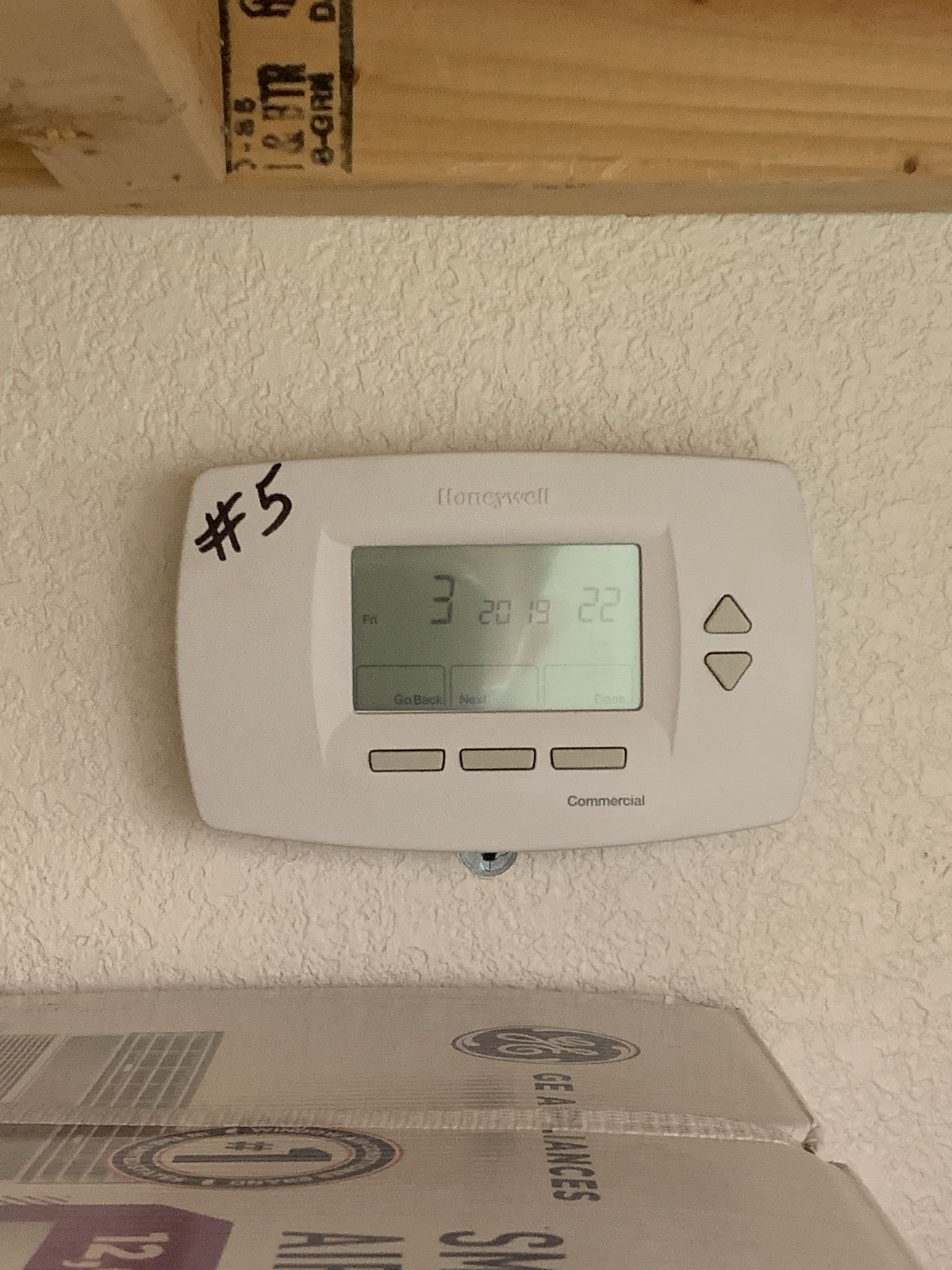The indoor photograph showcases a newly constructed interior space. Central to the image is a Honeywell thermostat, prominently featuring a black number 5 on the left side of its clean, white case. The device sports a digital display with grey buttons positioned on the right side for temperature adjustments. Additionally, three grey buttons are situated below the display, likely for changing operational modes. The thermostat is mounted on a white, textured wall. Near the bottom of the photograph, a cardboard box labeled "GE Appliances" is partially visible. The top portion of the image reveals unfinished wall studs, suggesting a stage of construction or renovation, with exposed 2x4 wooden beams.